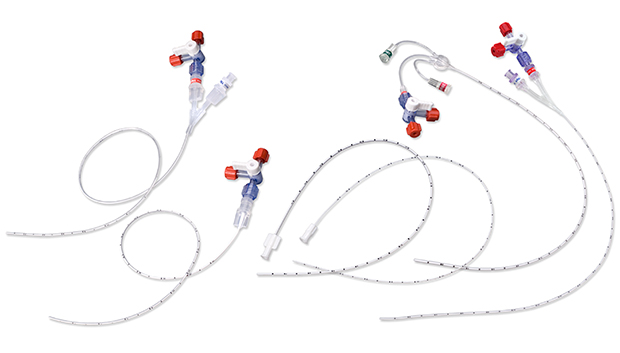The image showcases an array of fine, mostly clear medical tubes, reminiscent of those found in hospitals or doctor's offices, laid out on a pure white background, suggesting a catalog photograph. These tubes feature intricate components at their ends, including blue connectors and red knobs or caps. Some tubes split into multiple segments, with distinctive red caps at the terminations, while others are adorned with white plastic levers, resembling those used to control fluid flow, allowing for the increase, decrease, or cessation of movement through the tubing. Additionally, black markings can be observed at intervals along the tubing, and some components appear to be designed for insertion or connection to other medical apparatuses.